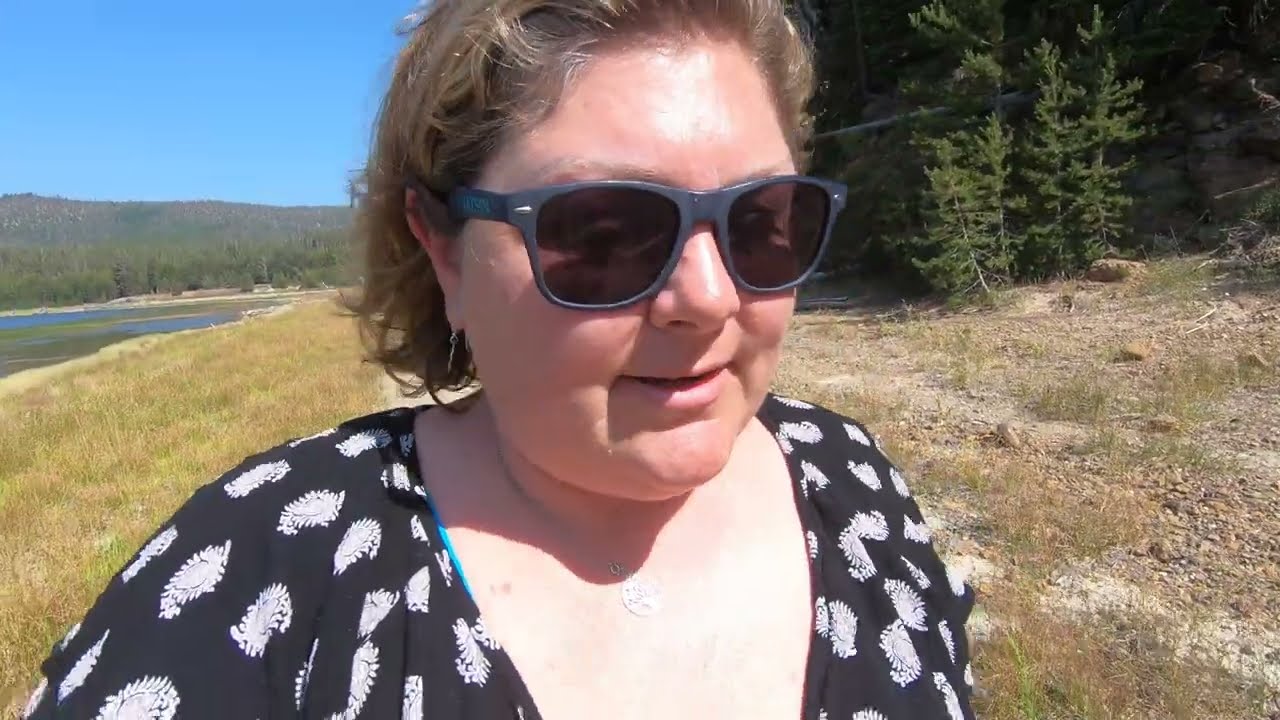The image captures a white woman, likely around 40 years old, from her chest up. She has sandy blonde or light brown hair pulled back from her forehead and is wearing dark black sunglasses with heavily tinted lenses. She dons a black v-neck blouse or dress adorned with a repeating small white design, complemented by a silver necklace. The woman, slightly heavy-set, is positioned in the central part of a rural outdoor setting. In the background, rolling hills or mountains can be seen in the distance, alongside a grassy, possibly arid, area with a dried-up pond or lake. Trees are visible to her right and left sides, with a clear, mostly blue sky overhead. The image is a horizontal rectangle, and the woman’s mouth is partially open, as if she is speaking. The main colors present in the photo are black, white, tan, beige, green, brown, gray, and blue.